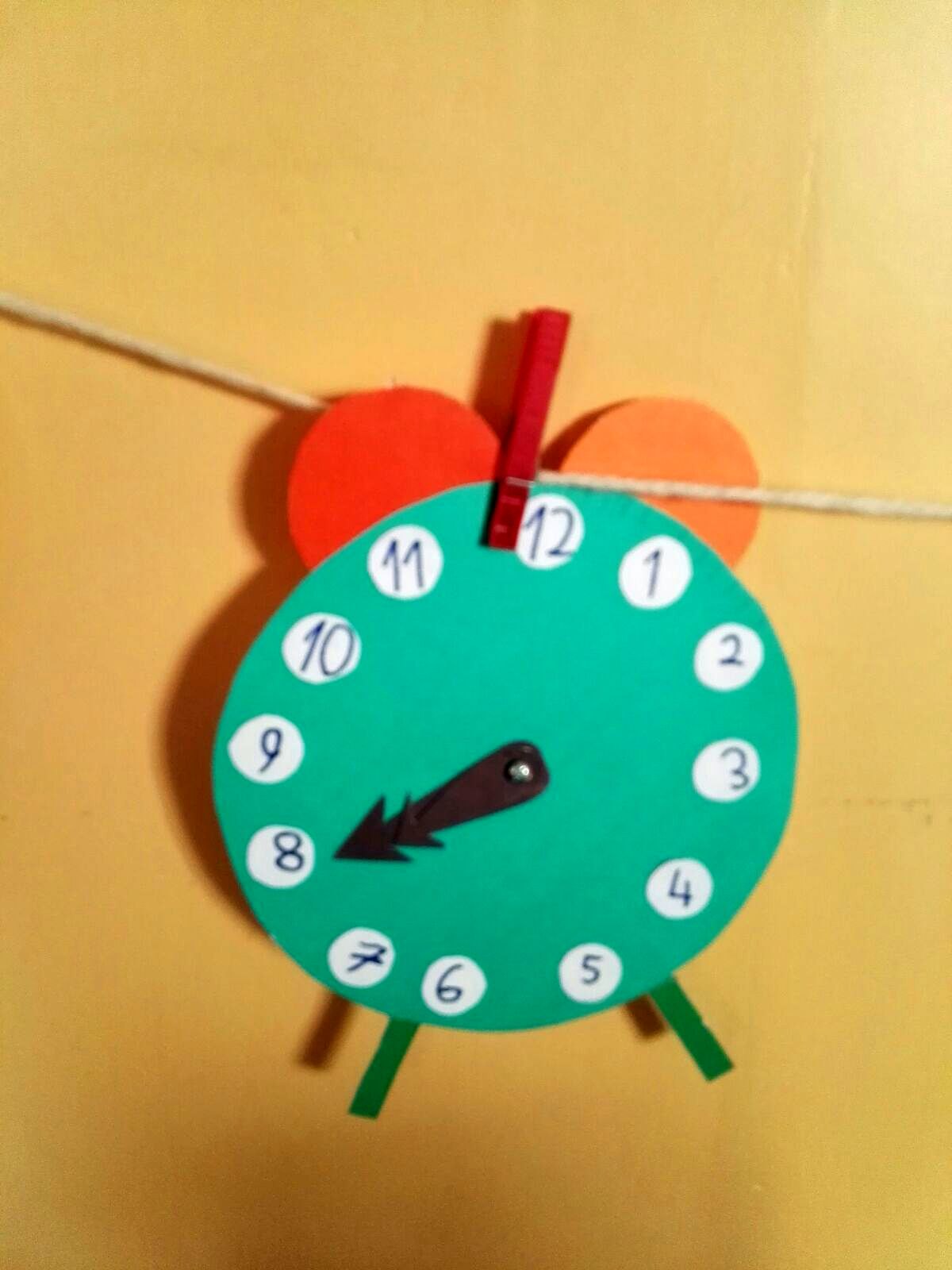This photograph features a handmade, non-functional analog clock hanging against a mustard yellow background, likely depicting a kindergarten classroom scene. The round clock face, which is light green, appears to be made from either paper or painted wood. It has numbers encased in white circles that resemble glued-on paper, with a distinctive European-style crossed seven. The black hour and minute hands are positioned to indicate 7:40. At the center of the clock is a silver pin securing the hands. Two green legs are attached to the bottom of the clock face, giving it a whimsical appearance. At the top, in the manner of Mickey Mouse ears, are two half-circles—one orange and one red. The clock is suspended from a piece of twine stretched horizontally, and a red wooden clothespin secures it to the twine.